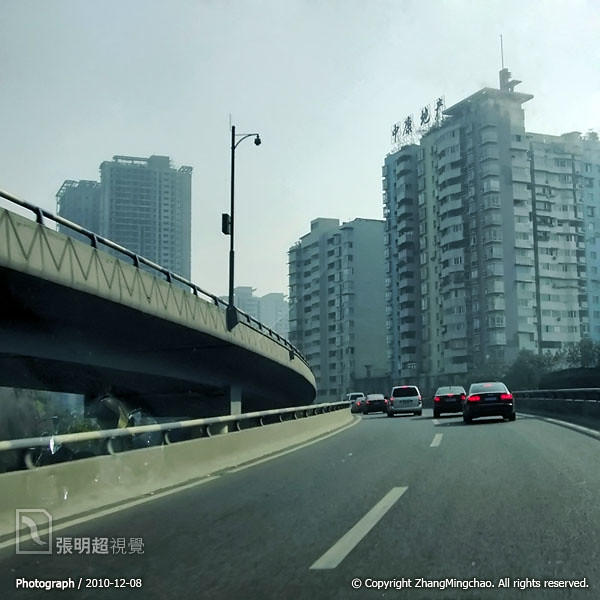This detailed color photograph from 2010 depicts an urban scene taken through a car windshield on a curved flyover ramp. The view showcases a busy highway with two lanes of traffic heading away from the camera, dominated by dark-colored vehicles. In the center left, another raised section of the highway is visible, featuring tall streetlights designed to illuminate both roadways. The infrastructure is surrounded by a mix of lush trees and towering skyscrapers in the background, which include residential and commercial buildings, one of which displays a large hoarding with Chinese characters.

The scene is illuminated under a clear, white day sky, adding a crisp contrast to the urban landscape. On the lower part of the flyover, prominent railings line both sides, demarcating the road. The photograph is marked with a distinct textual annotation; the bottom left reads "Photograph 2010-12-08" accompanied by a symbol resembling a snake, while the bottom right corner states "Copyright Zhang Mingchao, All Rights Reserved." The overall visual style of the photograph is representational realism, capturing the essence of the city's infrastructure and daily commute.